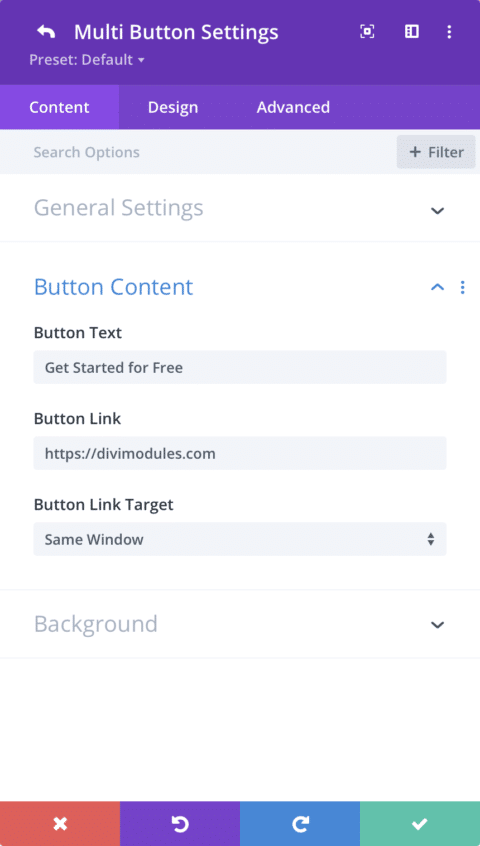The image depicts a detailed user interface of a software application, possibly related to web design or programming, specifically for configuring multi-button settings. At the top, a purple banner displays the headings "Preset Default," "Content," "Design," and "Advanced," accompanied by several icons. Below the banner, on a white background, there are various sections and configurable options for buttons. These include:

- **Search Options**: Arranged from left to right
  - **General Settings**: Where overarching button preferences are managed.
  - **Button Content**: For inputting the button's text, the example here is "Get started for free."
  - **Button Link**: containing a designated URL, in this instance, "DiviModules.com."
  - **Button Link Target**: Specifies the link behavior (here, it is set to "same window").
  - **Background**: Likely for altering the button or interface's background.

At the bottom, a palette showcases colors red, purple, blue, and green. The green section houses navigational icons: an "X" for closing, backward and forward arrows, and a checkmark for confirming settings. Additionally, "Filter" appears at the top right beneath the purple banner, likely to refine search or options within this interface.

The interface, with its comprehensive yet structured layout, suggests that it is a functional part of a web design or programmatic module configuration, emphasizing user customization through its segmented options and vibrant color codes.